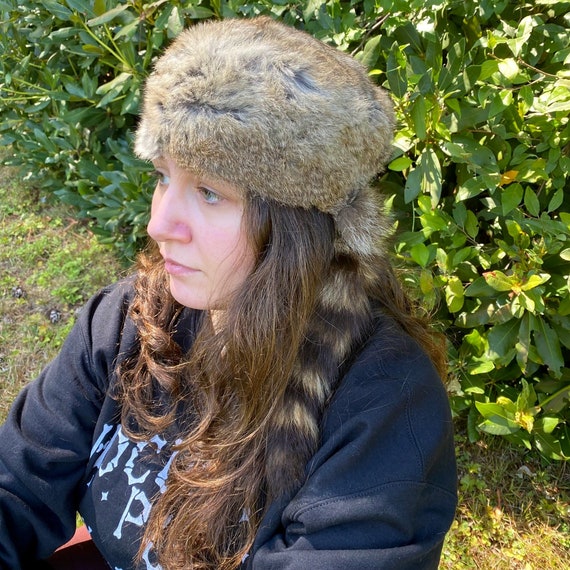This square photograph captures a young woman sitting outside on mowed grass with a slightly unkempt bush behind her. She wears a distinctive raccoon fur cap with the raccoon's tail draped over her long, wavy brown hair, which cascades both in front of and behind her shoulders. Her attire features a dark sweatshirt with some unreadable white text on the front, partially obscured by her hair. The woman has striking bluish-green eyes and a pensive expression as she gazes slightly to the left of the camera. Her cheeks and nose are slightly red, possibly from the cold, adding a natural blush to her complexion. The sunlight enters from the upper right corner of the image, highlighting her subtle lip gloss. Despite her thoughtful demeanor, the overall scene is bathed in gentle sunlight.